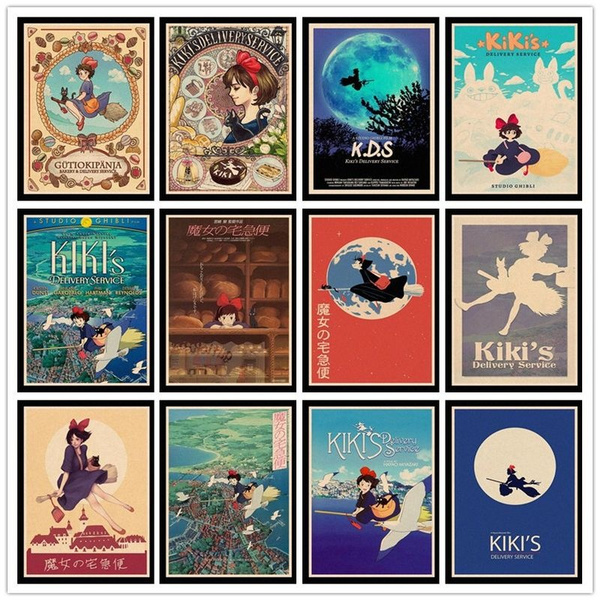The image features a collection of twelve vibrant and nostalgic advertisements depicting various scenes and promotional materials from the 1989 Japanese animated film "Kiki's Delivery Service," based on the storybook. The posters, arranged in three rows of four, each capture distinct moments involving the young witch Kiki, who is easily recognizable by her dark brown bob haircut, large red bow, long blue dress, red shoes, and reddish-orange handbag. The backdrop of many posters shows Kiki flying on her broomstick, often accompanied by her black cat, with several images prominently featuring the moon, reminiscent of the famous ET poster. The posters, which resemble stamps in size, predominantly feature Japanese text alongside the film's title in English, highlighting Kiki in various dynamic poses as she embarks on her aerial delivery adventures, emphasizing the film’s charm and appeal to children.